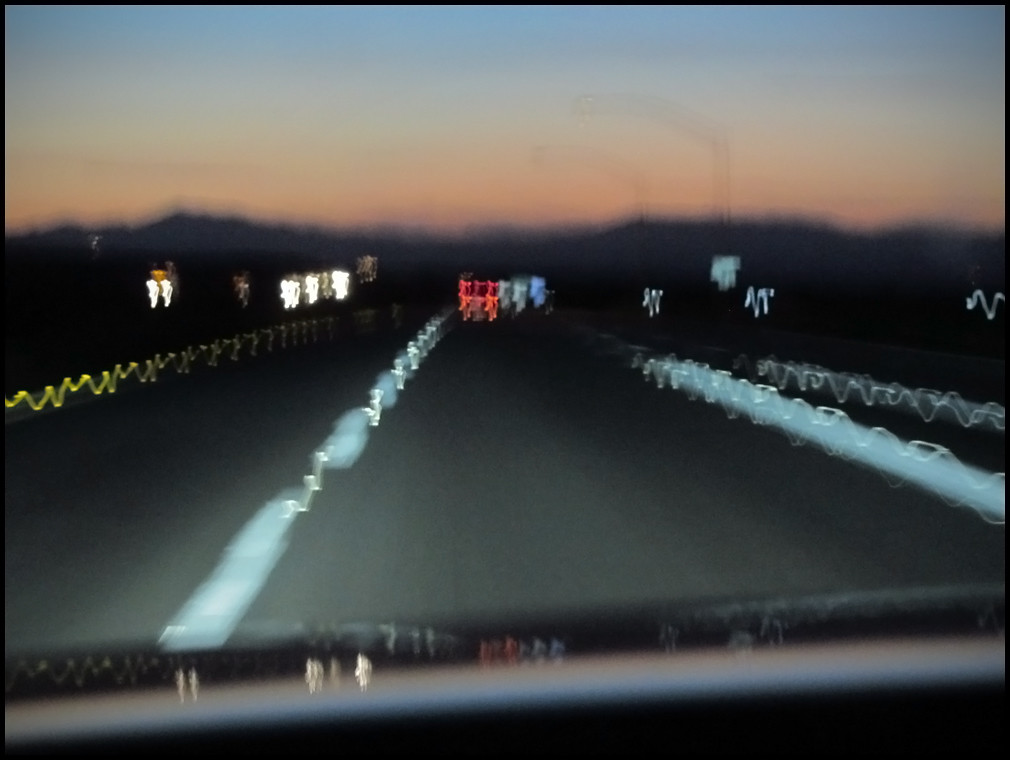Photograph Description: This image captures the view from the driver's seat of a moving car during dusk. The photograph is heavily distorted and blurred, creating an abstract portrayal of the scene. Street lines extend forward into the distance, guiding the viewer's eye down the road. In the background, the last rays of the setting sun linger on the horizon, signaling the transition into night. The blurred red brake lights of the cars ahead form wavy, squiggly patterns, enhancing the sense of motion. Similarly, the headlights of oncoming vehicles create wavy streaks of light, contributing to the overall surreal quality of the image. The interplay of the blurred lights and the twilight sky provides a captivating, almost dreamlike atmosphere, making the distorted lighting the primary focal point of this photograph.